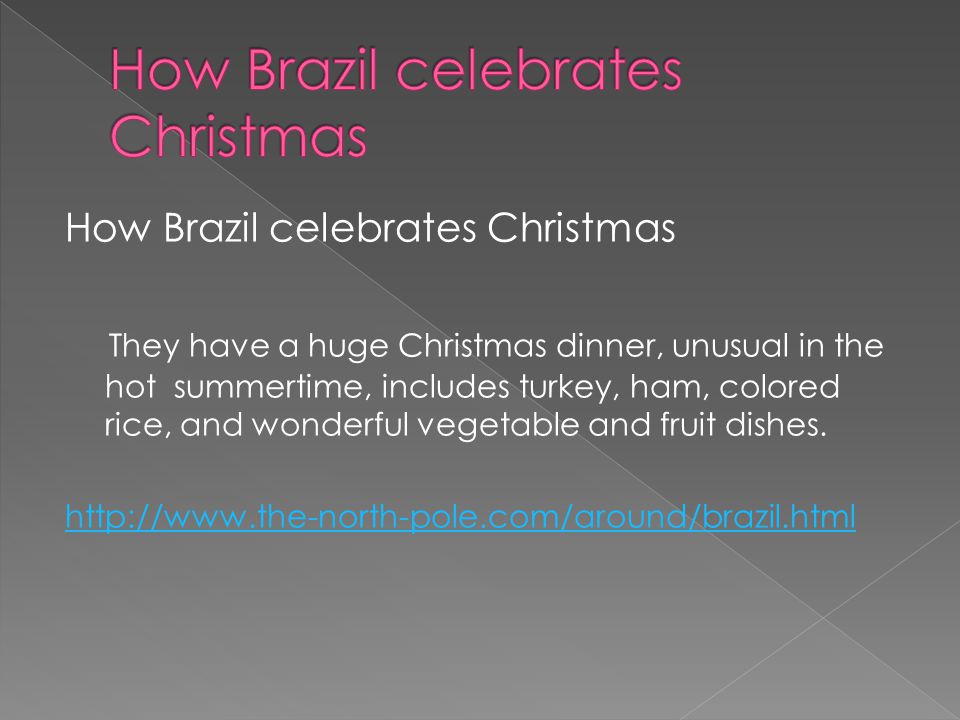The image features a text on a dual-toned grey background, divided diagonally by a thin line running from the top left corner to the bottom right. The top right section of the background is a dark grey, while the bottom left section is a light grey. 

At the top of the image, there is a prominent pink text that states, "How Brazil Celebrates Christmas." Below the pink text, the same statement is repeated in white. 

At the bottom of the image, additional white text reads, "They have a huge Christmas dinner unusual in the hot summertime. Includes turkey, ham, colored rice, and wonderful vegetable and fruit dishes."

A blue, underlined URL is positioned at the very bottom, providing further information.